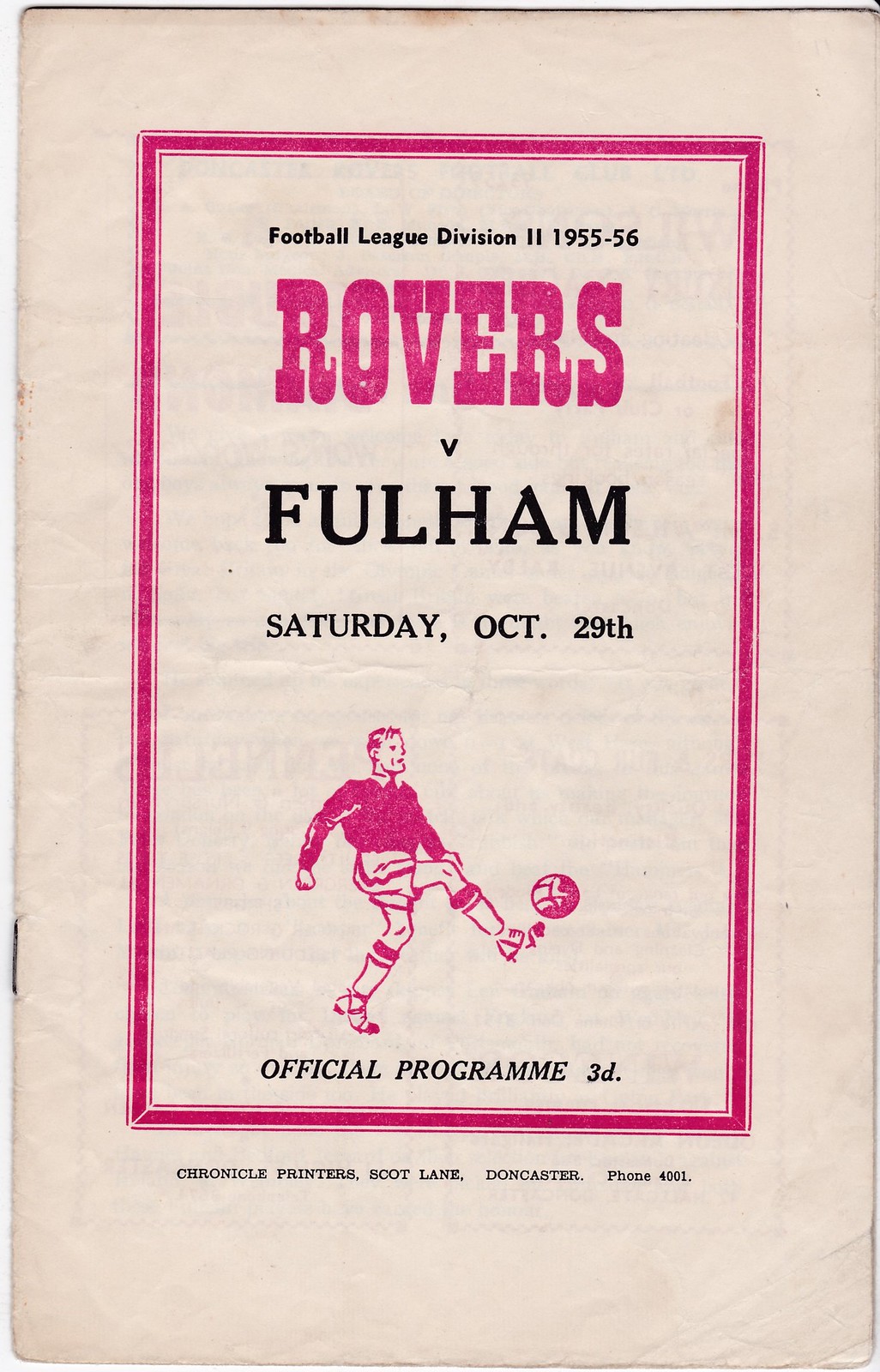The image is a vintage soccer program cover printed on off-white paper with a red rectangular border. The text predominantly features shades of red and black. At the top, in large red font, it reads "Football League Division 2, 1955-56." Below, it states "Rovers vs. Fulham, Saturday, October 29th," with a note of "Official Program, 3D" printed underneath in black. The cover displays a red graphic of an Englishman wearing a dark jersey, light shorts with a red stripe, and knee-high socks, mid-action kicking a soccer ball. Additionally, the bottom provides small, black printed text reading "Chronicle Printers, Bolt Lane, Doncaster, phone 4001." The print's light pinkish background and visible staples suggest it’s a booklet rather than a single page, preserving its historical essence from the 1955-56 football season.